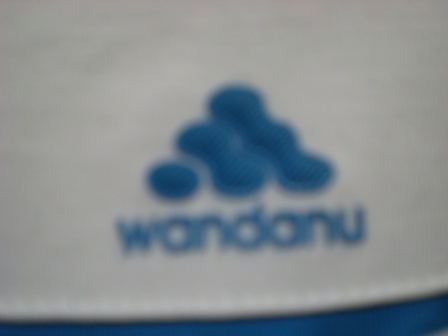This digital photograph captures an extremely close-up and somewhat blurry view of an object, likely a fabric surface, characterized by a predominantly white or whitish-gray background. The photo is landscape-oriented, and at the bottom portion of the image, there's a darker blue streak that rises towards the right, suggesting a possible curve or stitching, which might indicate it's an item of clothing, possibly a cap or hat. Central to the image is the logo of the brand "WANDANU," consisting of a slightly obscure blue text written in a rounded, somewhat stylized font. Above the lettering, a design featuring six dark blue circles is arranged. The circles are organized in a formation that resembles a pyramid or triangular stack: one circle at the top, two directly below it linked by a notch, and three at the base, also linked by notches. Despite the blur, the logo and brand name are distinctly blue, emphasizing their prominence against the lighter background.